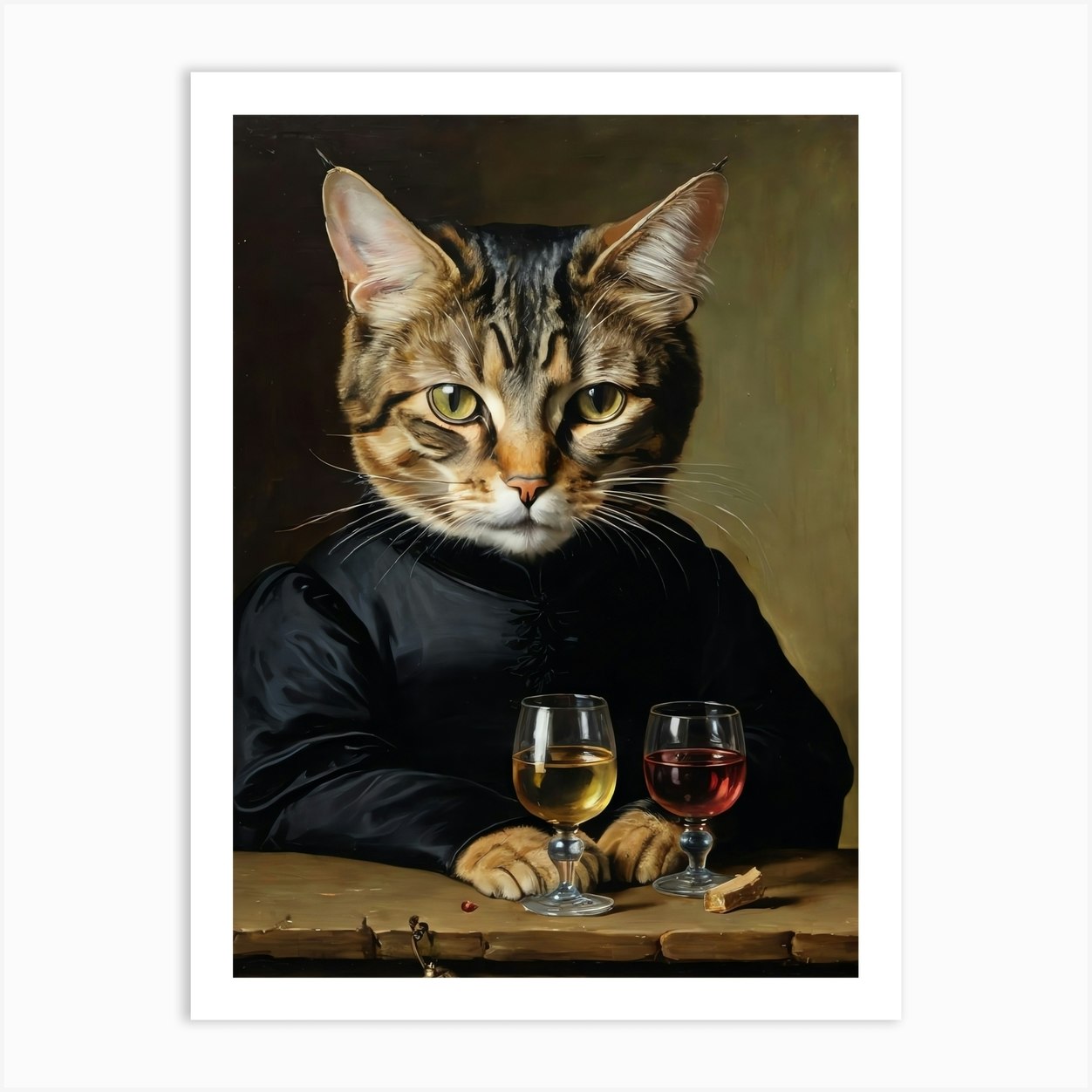The image depicts a detailed and surreal representation of a cat that resembles a tiger, with distinctive stripes and a combination of blonde, dark, and brown fur. The cat is notably wearing a black, long-sleeve satin shirt with puffy shoulders and laced front. It has expressive green eyes, and its nose and mouth area are white with a pink nose. The cat appears to be seated at a stone-like table, with its furry paws notably touching two wine glasses—a taller one containing white wine and a shorter one with a red or rosé wine. There seems to be an additional, somewhat ambiguous object next to the glasses, possibly a piece of cheese. The background is a muted olive and brown, and the entire image is framed on a piece of white paper, with a shadow suggesting it's placed on another white surface. The artwork has the smooth texture often associated with AI-generated images, enhanced by an impression of an oil painting. The cat's serious expression is directed towards the viewer, adding an intriguing focal point to the composition.